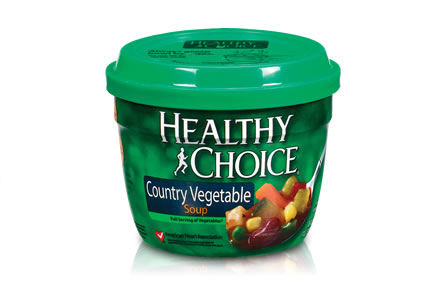The image features a vibrant green microwaveable food container topped with a removable plastic lid. The lid sports a prominent black rectangle with minuscule black text. Directly below this, the words "Healthy Choice" are prominently displayed, accompanied by an illustration of a white silhouette of a person running. The label indicates that the flavor is "Country Vegetable Soup." Adjacent to this, an appetizing depiction showcases pieces of zucchini, carrots, and corn elegantly arranged within a silver spoon. Additionally, a small red square with a white check mark is situated towards the bottom left corner of the container. The overall height of the soup container is approximately five inches.